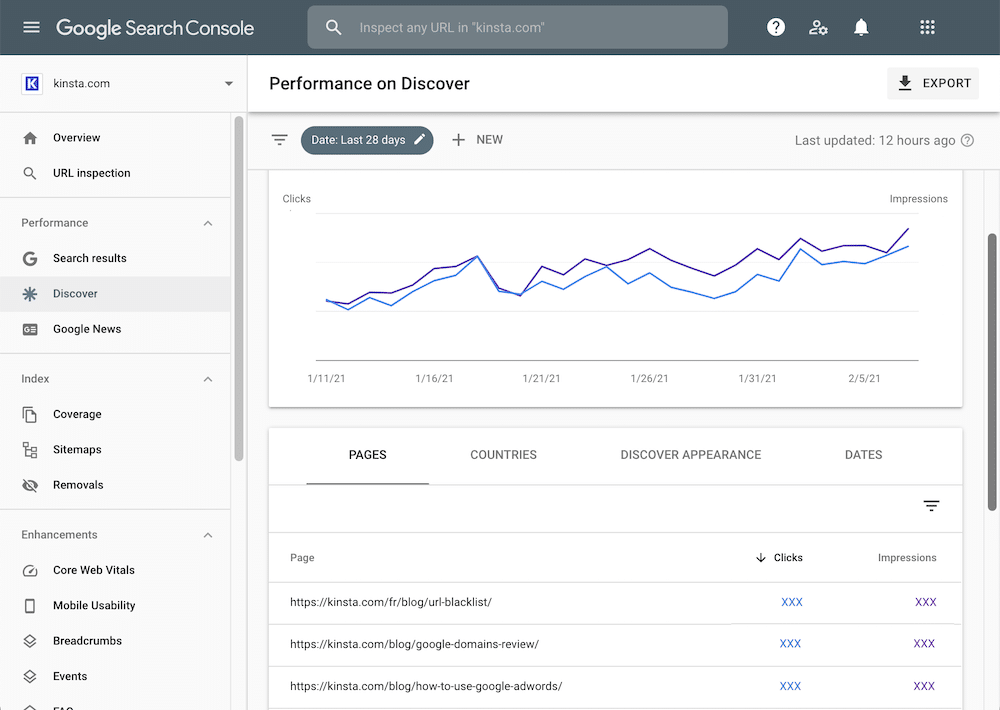This screen capture is from the Google Search Console website. At the top of the image, there is a gray toolbar featuring a menu icon composed of three horizontal lines on the far left. Next to it, the text "Google Search Console" is displayed. Centrally located within this toolbar is a lighter gray search bar with the placeholder text "Inspect any URL in kinsta.com." To the right of the search bar, there are several icons: a question mark within a circle, an account icon coupled with a settings gear, a bell, and a grid menu icon.

Beneath the toolbar, on the left side of the screen, there is a vertical pull-out menu offering various navigation options. The main section of the screen displays detailed information pertinent to the website's performance. At the top of this section, the text "Performance on Discover" is shown on the left, while an "Export" option is available on the far right.

A central graph visually represents the number of user clicks on the website over a designated period, spanning from January 11, 2021, to February 5, 2021. Below the graph, there is a segmented breakdown of the website's performance metrics, including pages, countries, discover appearance, and dates, allowing users to edit and refine their website data and performance analysis.